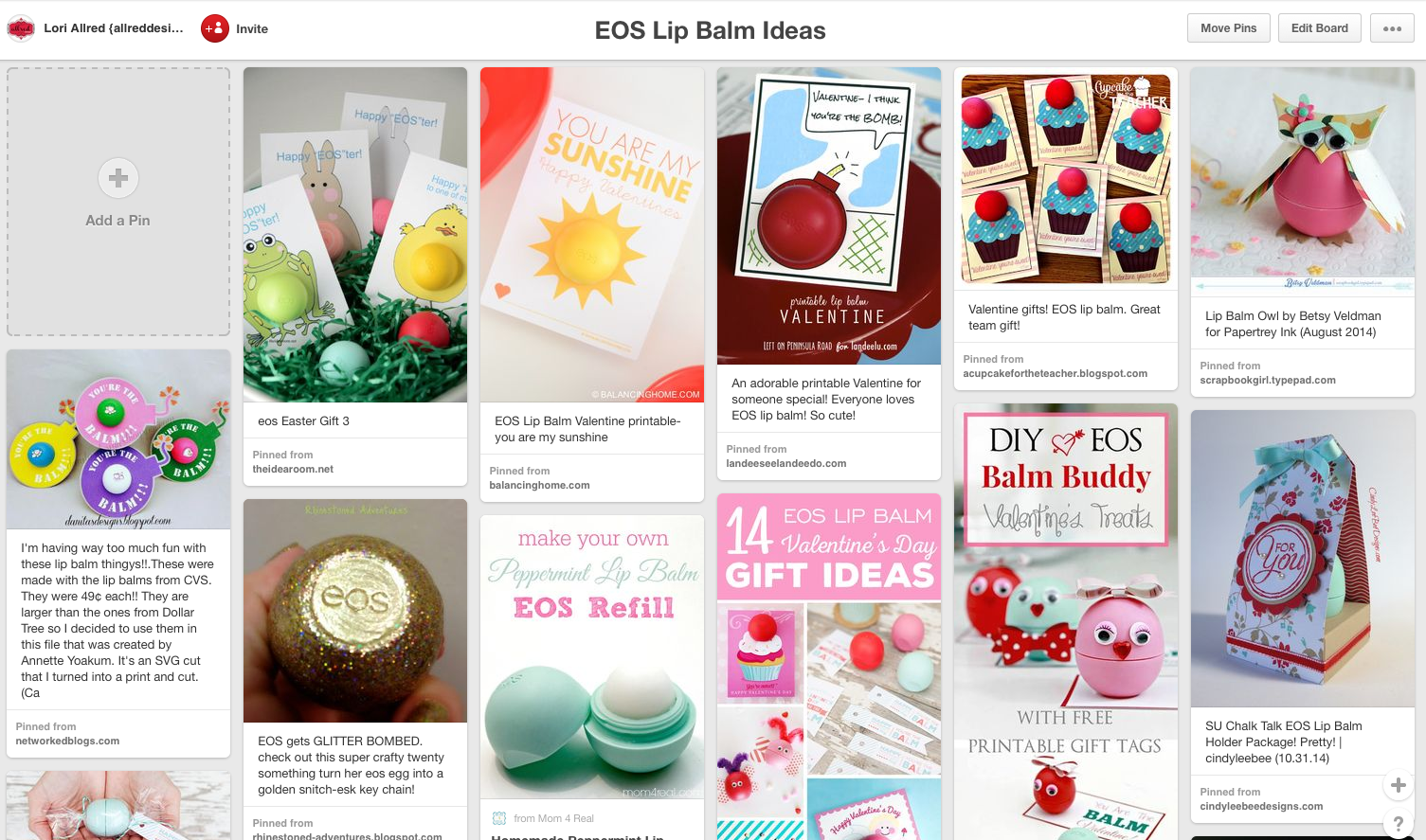This screenshot showcases a Pinterest board curated by a user named Lori, identifiable by the little red icon in the upper left corner. The user has named this board "EOS Lip Balm Ideas," reflecting a collection of creative uses for EOS lip balm containers, which are known for their distinctive, unscrewable, Easter egg-like design with a soft, spherical balm center.

On the upper right, there are functional buttons labeled "Move Pins," "Edit Board," and a button represented by three dots for additional options. The board is organized into a grid of six rectangles across and two columns down, making a total of twelve slots. The top-left slot remains empty with a prompt to "Add a Pin."

The pins on this board exhibit various innovative ideas. For instance, the second pin on the top row shows an EOS lip balm incorporated into an Easter basket as an Easter egg. Another creative pin on the upper right corner features a lip balm designed to resemble an adorable owl, crafted by Betsy Veldman for Papertree, Inc., dated August 24th. This whimsical design includes a pink EOS balm embellished with decorative wings and a bird mask.